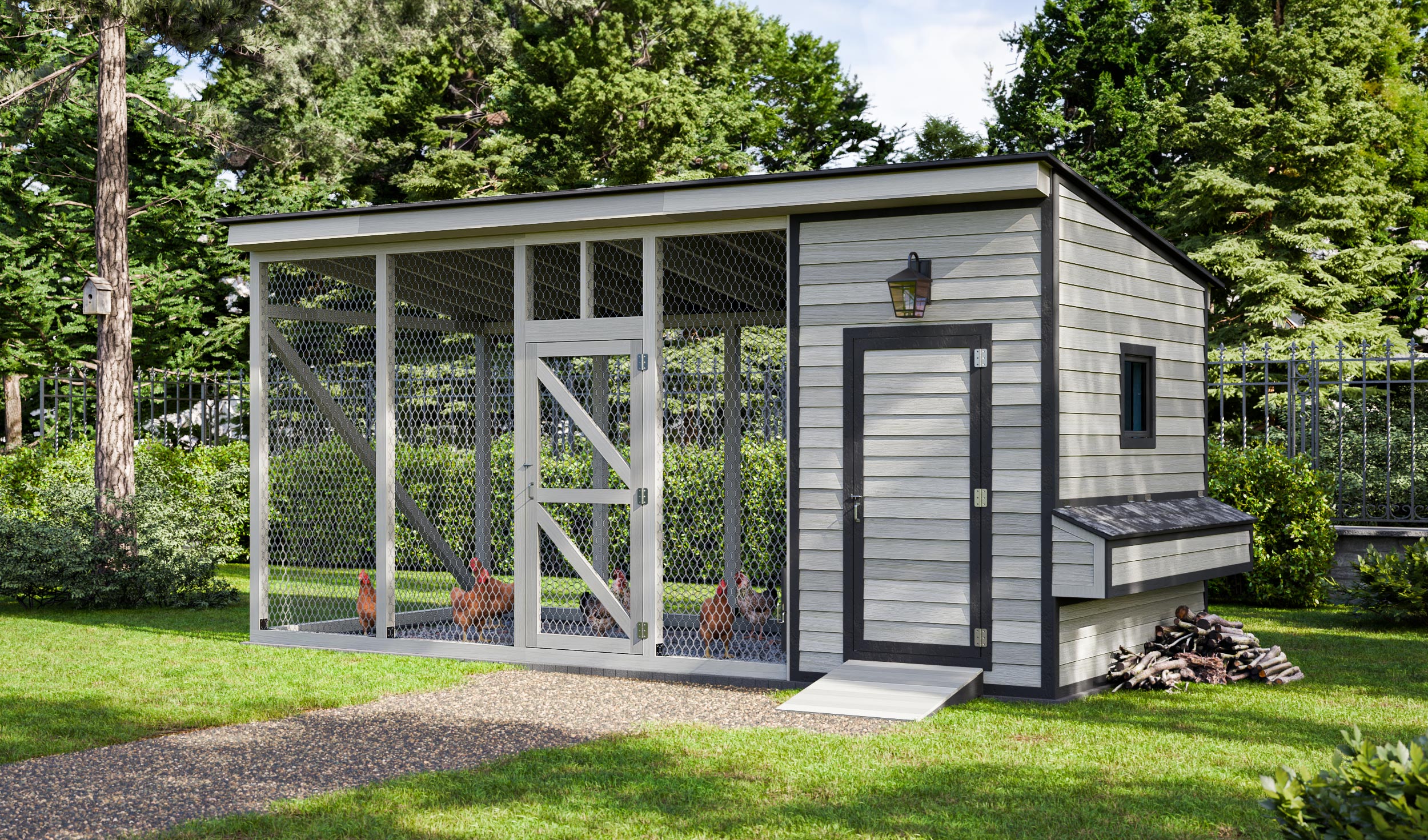A picturesque scene unveils a meticulously maintained chicken coop nestled right outside a house, set against a backdrop of towering trees. This coop presents itself as a gray and white wooden structure, exuding a sense of sophistication uncommon to typical coops. The right side of the coop is enclosed and features a full-sized door with a dark brown frame and silver hinges, complemented by a hanging lantern that remains off in the early morning light. A gravel sidewalk leads visitors to a small concrete slab before the door, surrounded by lush green lawns and a scattering of firewood beneath an overhang for protection.

The main body of the building is bordered with a chain-link fencing that is held together by horizontal and diagonal planks, providing an open view of the interior. Inside, a mix of orangish-red roosters and hens are visible. An additional ramp at the entrance offers easy access for the chickens. The entire set-up, right down to the smallest detail of stacked firewood on the side, speaks to a high-class, thoughtfully designed coop within a serene and picturesque yard.